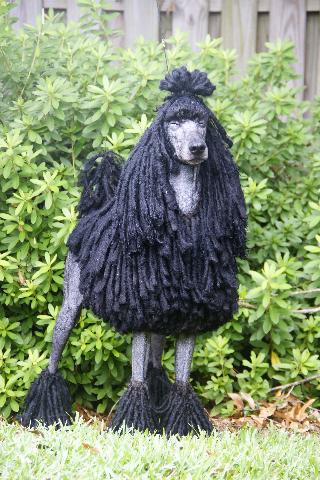In this photograph, a strikingly groomed standard poodle is featured standing on a well-maintained green lawn scattered with a few brown leaves. The dog, with its distinctive black dreadlocked coat, conveys an air of sophistication and meticulous grooming. The fur on its head forms a neat poof, tied back smoothly, while its face and neck are clipped close to the skin, revealing a gray skin tone. Each leg is similarly clipped, exposing the skin, but the fur at its ankles forms elegant, long, string-like tufts. The background showcases a lush green bush with small, fanning green and yellow leaves, adding a vibrant contrast to the scene. Behind the bush, a light gray wood fence with vertical planks adds depth to the composition. The poodle stands alert and poised, its eyes seemingly closed and its black nose prominent, creating a charming and picturesque tableau.